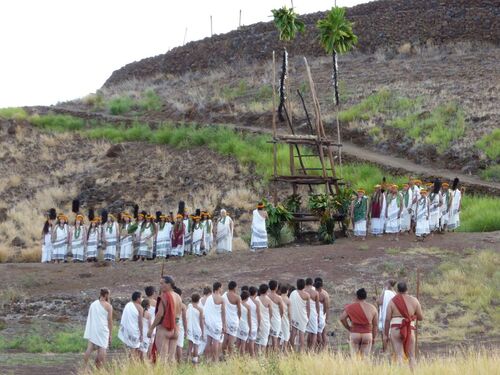The photograph depicts a significant scene set against a barren, rocky, and grassy landscape with a couple of palm trees and a conspicuous wooden ladder in the middle. The sky above is clear and pale, suggesting either early evening or late afternoon. There are two distinct groups in the image, both clad in traditional white garments. The group further away seems to consist primarily of women adorned with green floral leis, while the nearer group appears to be composed of men, some of whom wear white short togas with one shoulder exposed and red scarves tied around their torsos. The men are standing on a patch of yellowing grass, while the grass near the women looks greener. Both groups face each other, creating an impression of a ceremonial or tribal gathering. The overall atmosphere suggests an important event possibly of a religious or cultural nature, with all participants appearing to be deeply engaged in the proceedings.